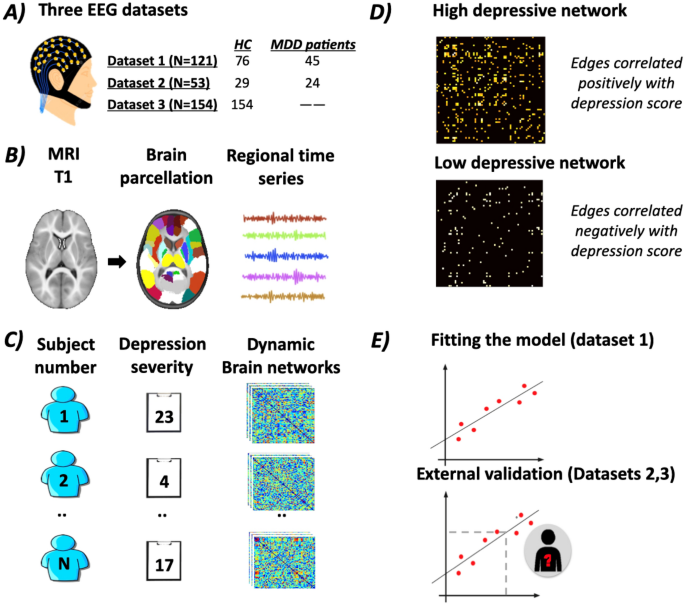This image is a detailed, computer-assisted display explaining how MRI data can be used in the study and treatment of depression. The diagram is divided into five sections labeled A through E, each representing different data sets and visualizations.

- **Section A**: Features a human figure wearing a black cap, labeled "three EEG data sets." This section includes a chart that is predominantly black.
  
- **Section B**: Provides MRI images and brain parcellation figures. A concise three-column layout showcases a black and white brain image, a colorful brain image with labels like MRI, T1, regional time series, and color bars in red, green, blue, purple, and orange.

- **Section C**: Focuses on subject numbers, displaying a three-column by four-row grid. The first column contains icons of blue human figures, the second column lists specifics in white and black rectangles, and the third column features multicolored charts representing dynamic brain networks.

- **Section D**: Contains two sections highlighting network photos, showing 'high-depressive network' and 'low-depressive network' data blocks. It differentiates agents positively and negatively correlated with depression scores.

- **Section E**: Features line graphs positioned to reveal fitting models of data sets. The top graph represents data set 1 while the bottom graph offers external validation for data sets 2 and 3. The bottom graph includes dotted lines and an icon inset with a question mark, indicating an area for further investigation or ambiguity.

This comprehensive diagram effectively uses visual aids to present various forms of neural data analysis and their implications for understanding and treating depression.